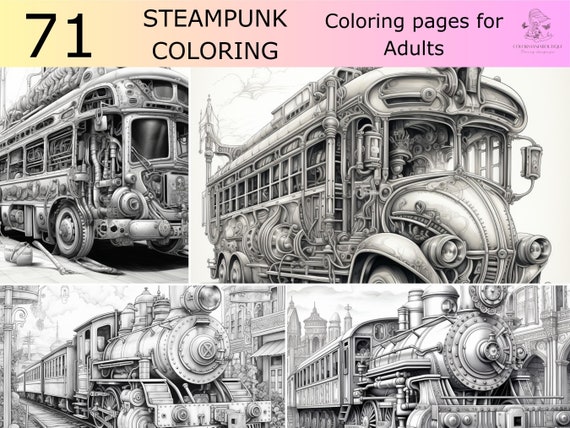The image is a promotional cover for a steampunk-themed adult coloring book titled "71 Steampunk Coloring: Coloring Pages for Adults." The banner at the top transitions from peach yellow on the left to light purple on the right, featuring bold black text with the book's title and a small, illegible purple logo at the far right end. Below this banner, the image displays a grid of four intricate black and white line art illustrations designed for coloring. The top left image depicts a large industrial bus with a flat front, while the top right shows a similar bus but with a rounded, VW Bug-like front. The bottom left image features a detailed locomotive train with several attached cars, and the bottom right shows another train, this one slightly more detailed but with only one car attached. All illustrations are highly detailed with extensive industrial designs characteristic of the steampunk genre.